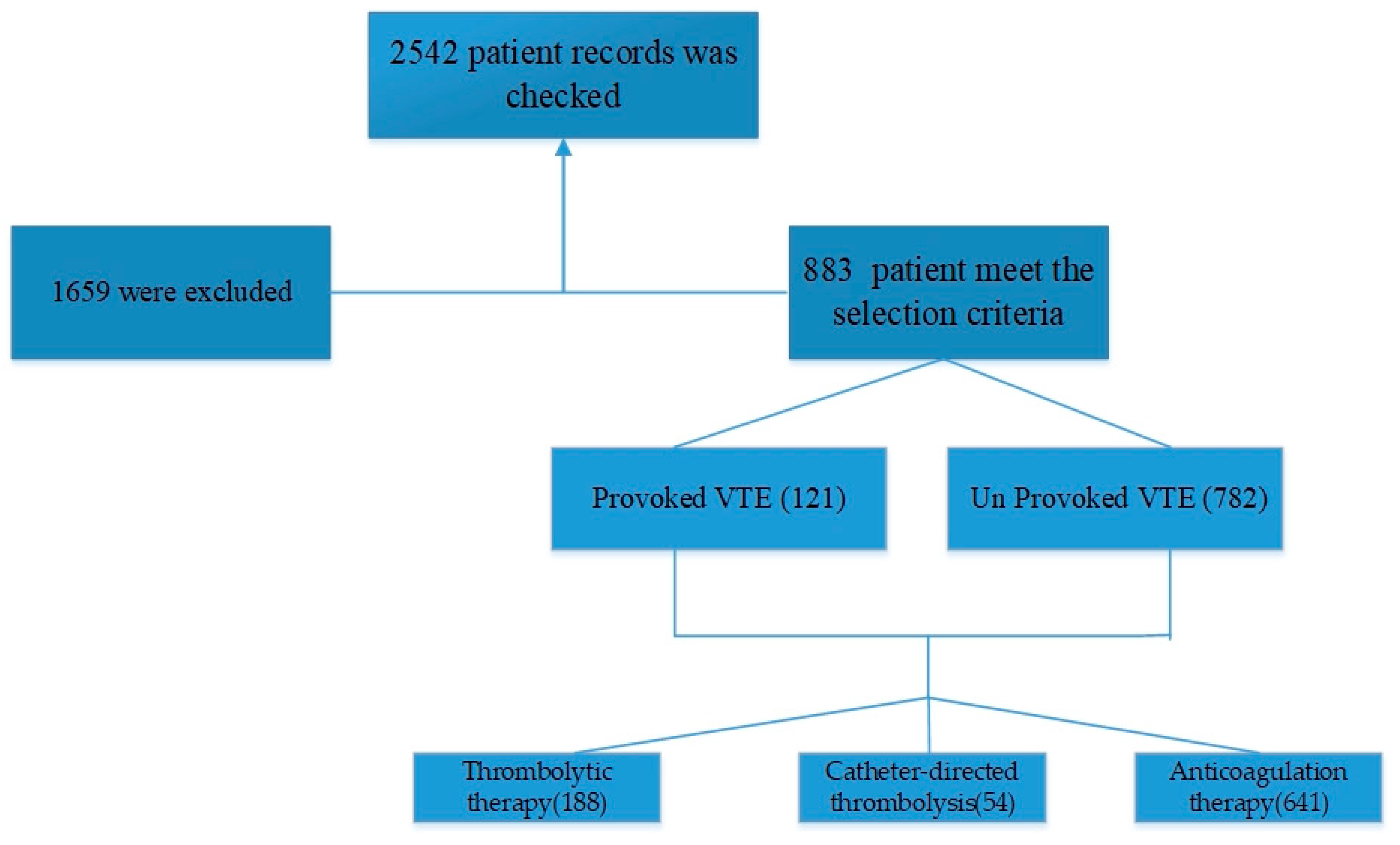This image is a detailed infographic in the form of a flowchart, featuring a white background with blue rectangular boxes connected by arrows that map out a selection process in a medical study. At the top, the chart begins with "2,542 patient records were checked" in black text inside a blue box. From these records, it notes that "1,659 were excluded" and "883 patients met the selection criteria." Moving downward, from the 883 patients, the flowchart divides into two categories: "provoked VTE" with 121 patients and "unprovoked VTE" with 782 patients. Further branching down, the chart details the subsequent therapies these patients received: "thrombolytic therapy" for 188 patients, "catheter-directed thrombolysis" for 54 patients, and "anticoagulation therapy" for 641 patients. The layout and color scheme suggest it could be created using Microsoft Office tools, aimed at explaining a medical study's methodology.